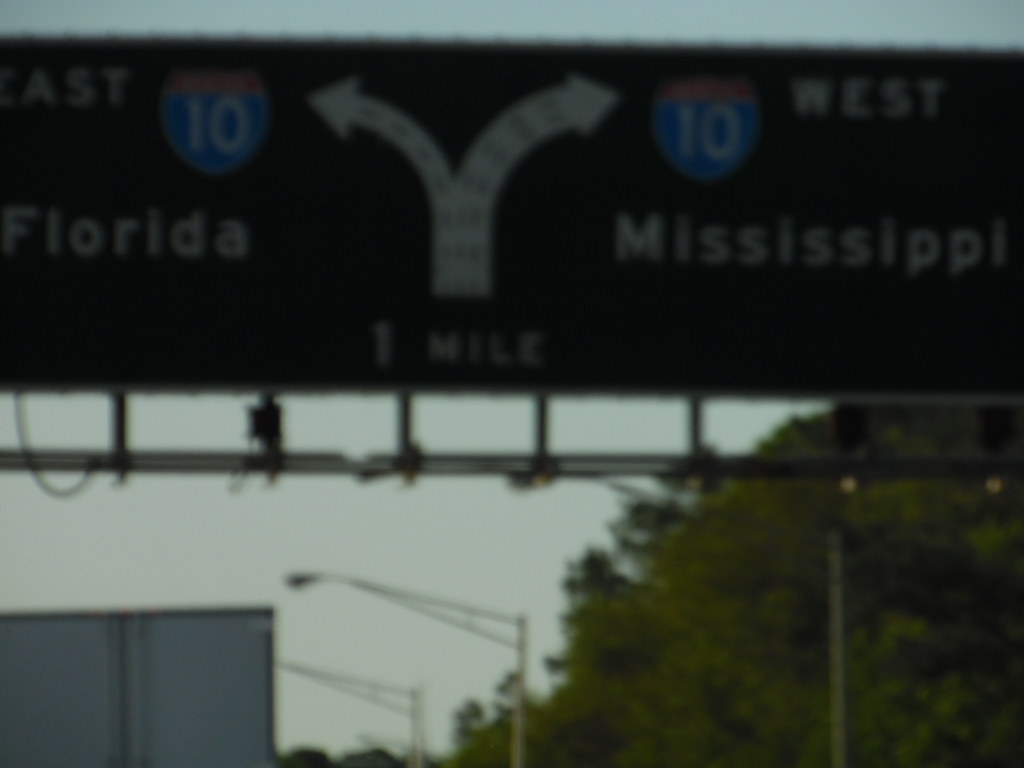The photograph, presumably taken from inside a car on a major U.S. highway, captures a cloudy gray sky as its backdrop. A row of trees begins at the bottom right corner, running parallel to a series of light poles. Dominating the top half of the image is a green highway gantry sign with white arrows pointing left and right. The arrows, extending from a central stubby white block, indicate directions for Interstate 10: "East Interstate 10 Florida" on the left and "West Interstate 10 Mississippi" on the right, both with their respective shields bearing a blue bottom and a red top. Beneath the interstate numbers, the sign states that the junction is one mile ahead. In the lower left corner, the image includes the back of a white semi-truck trailer, emphasizing the highway setting. However, no other vehicles are visible, suggesting the photo is angled slightly upward. The scene is framed with the route lined by trees and streetlights, reinforcing the impression of a broad, open road.